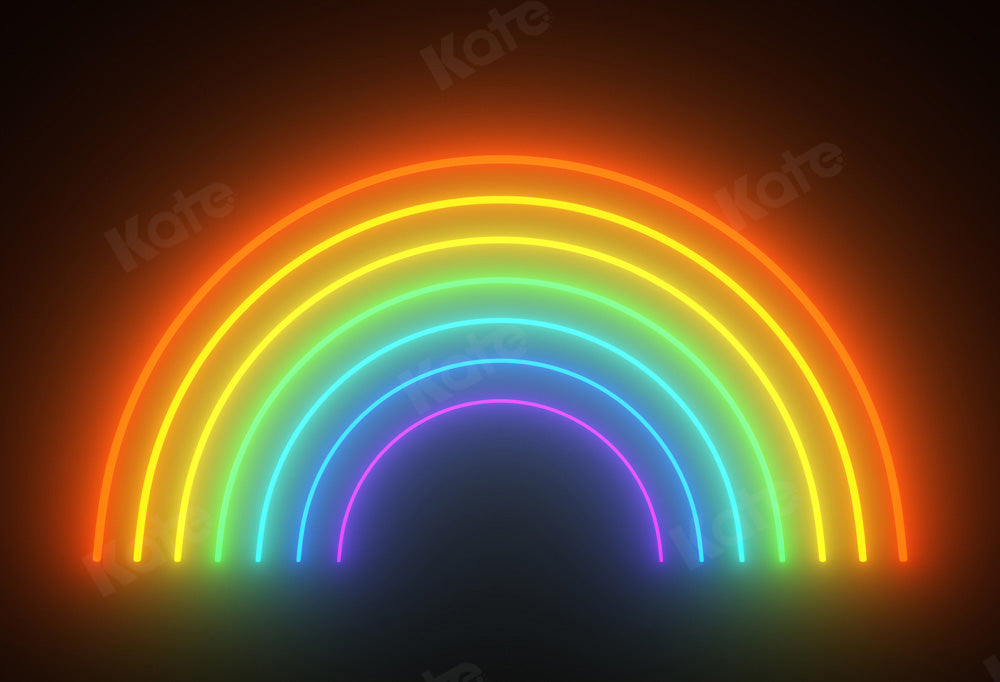The image is a rectangular digital stock photograph featuring an illuminated rainbow composed of neon lines, set against a stark black background. The rainbow arcs from the bottom left to the top right corner and comprises seven glowing, non-touching lines. From the outermost to the innermost lines, the colors are as follows: orange, yellow, another yellow, green, blue, another blue, and finally purple. Each of these vibrant neon lines emits a radiant glow that subtly overlaps with adjacent colors, creating a captivating ambient light effect. Overlaying the entire image diagonally, from the lower left to the upper right corner, is faded gray text that repeatedly spells out "Kate" (K-A-T-E), providing a textured overlay without distracting from the vivid neon rainbow.